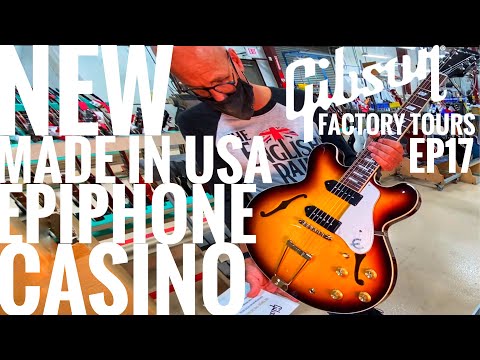This image is a detailed advertisement for the Gibson Factory Tours, Episode 17. The photo is framed with black bars at the top and bottom, creating a distinct banded effect. It features a bald man with a substantial brown beard, wearing glasses and a face mask. He's prominently holding an electric guitar with an orangey sunburst pattern, accentuated by a black outline and white elements near the strings. The man is wearing a shirt that has black sleeves and a gray torso with partially obscured text. The visible part of the shirt reads "The English R.A." and it features a British flag, the Union Jack, in a dome shape design. The background is somewhat indiscernible, but it hints at a shop, possibly a record store.

Overlaying the image are large, blocky white texts on both sides. On the left, it says, "New, Made in USA, Epiphone Casino." On the right side, in a more stylized angle, it reads, "Gibson" with "Factory Tours, Episode 17" in smaller blocky white text beneath it. The image likely serves as a thumbnail or promotional material for the Gibson Factory Tours, focusing on showcasing the guitar and the featured episode.